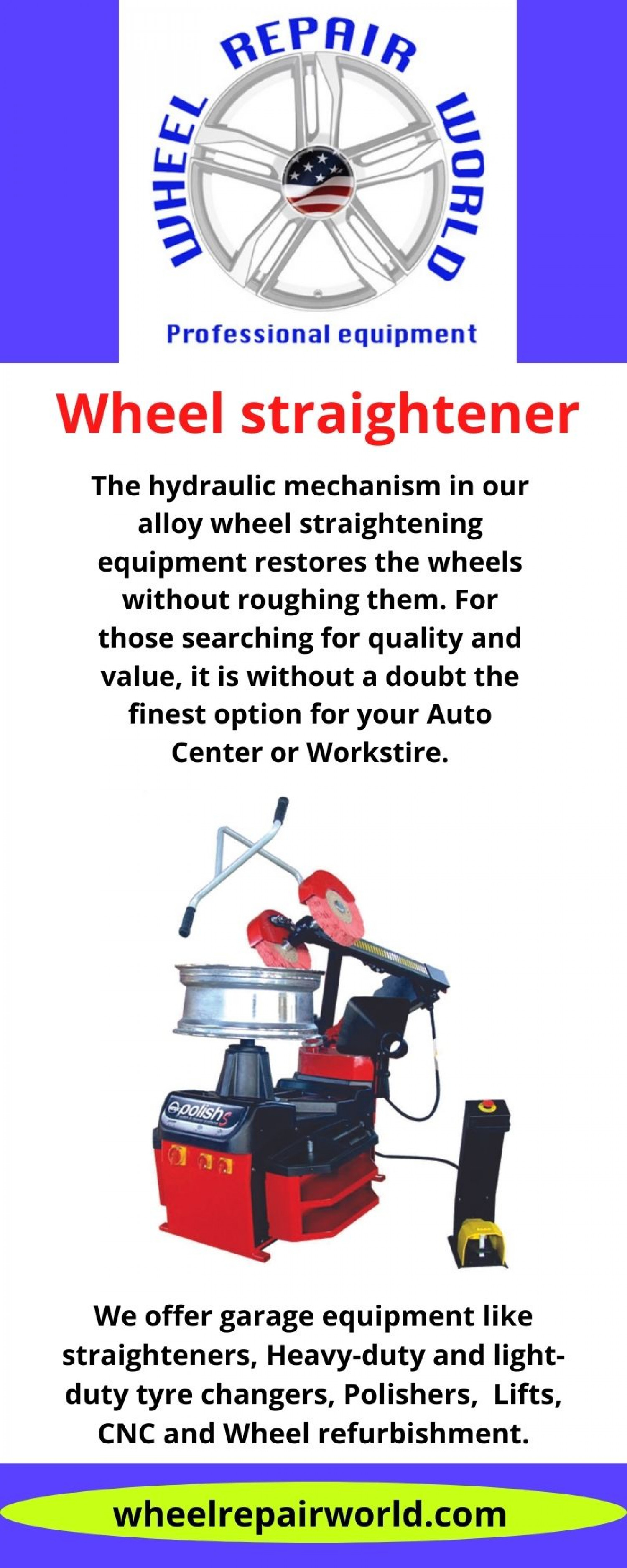The image appears to be the front portion of an advertisement or pamphlet for "Wheel Repair World." At the top center, a steering wheel prominently displays the American flag with blue and white stars on top and white and red stripes below. Encircling the wheel, in red text, it reads "Wheel Repair World," and beneath that, in smaller blue font, it says "Professional Equipment." Centered under this, in red font, is the term "Wheel Strictener," followed by a description in smaller black font: "The hydraulic mechanism in our alloy wheel strengthening equipment restores the wheels without roughing them. For those searching for quality and value, it is without a doubt the finest option for your auto center for work style." Below this description is an image of the red and black hydraulic machine with a silver circular container, presumably where the wheel is placed. At the bottom of the image is the website, "WheelRepairWorld.com."